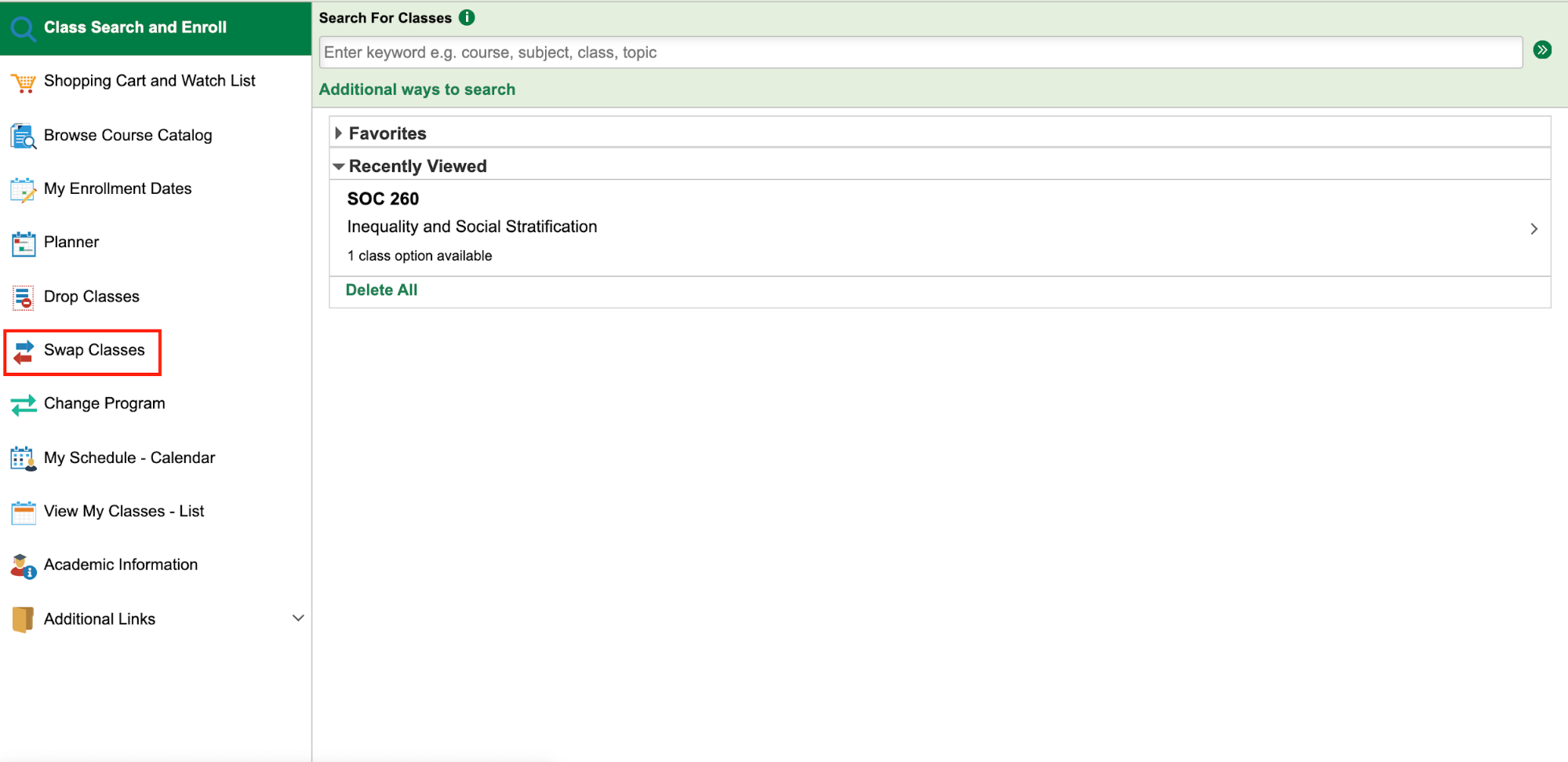The image displays a college course enrollment interface. In the top left corner, there is a green section labeled "Class Search Handle." Below it, a grey bar invites users to "Search for Classes" with placeholder text suggesting users can enter keywords such as course, subject, class, or topic. 

Further down, there are additional search methods and a section for "Favorites" as well as "Recently Viewed" items. Listed under this is "SOC 260: Inequality and Social Stratification," indicating one class option available. Next to it are buttons to "Delete All" and another labeled "Class Search and Enroll," located at the top left.

On the right side of this section, the interface consists of options such as "Shipping Cart," "Watch List," "Browse Course Catalog," "My Enrollment Dates," "Planner," "Drop Classes," "Swap Classes," "Change Program," and "My Schedule Calendar." There are also features to "View My Classes Dash List" and access "Academic Information."

In the "Swap Classes" section, there is a bidirectional arrow pointing left and right, encased in a red border, indicating the function allows students to swap classes. The overall layout includes multiple information boxes and symbols, suggesting a comprehensive college course catalog and enrollment system.